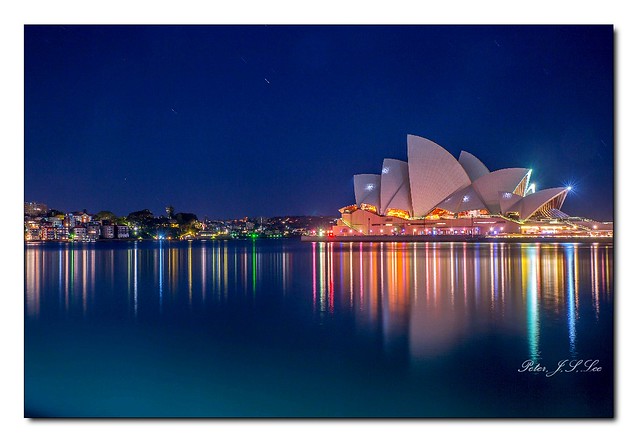The image depicts a striking nighttime scene of the Sydney Opera House, a radiant white structure with multiple angled facets, vividly illuminated against a twilight blue sky. In the right-center of the photograph, the Opera House stands prominently, while the left-center showcases commercial or residential districts of Sydney, with their myriad illuminated buildings. The varied colorful lights—blues, yellows, greens, reds, and pinks—reflect off the water in front, creating a breathtaking effect of elongated, multicolored streaks that resemble stalactites. This high-quality photograph, reminiscent of a postcard, captures the vibrancy and architectural splendor of Sydney. The photo is credited to Peter F. J. Lee, whose name appears in the lower right corner.